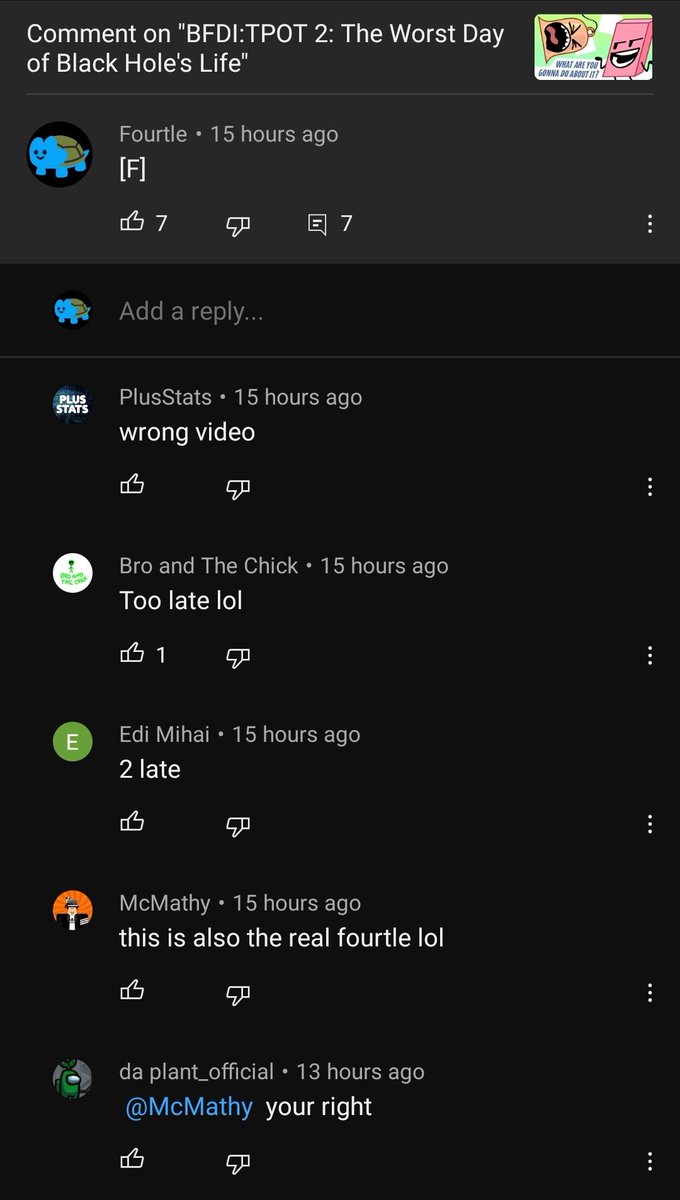This is a detailed screenshot of a mobile device displaying a black screen with a series of six comments on a video titled "The Worst Day of Black Hole's Life." The platform on which this video is hosted is not identified, as the app's interface and branding are not visible. 

1. The first comment is by a user named Fortal, who succinctly wrote "F."
2. The second comment, from Plus Stats, states "Wrong Video."
3. Following that, a user identified as Bro and the Chick commented, "Too Late LOL."
4. The fourth comment, echoing the previous sentiment, simply reads "Too Late."
5. Next, another entry claims to be from "the real Fortal," asserting "This is also the real Fortal."
6. Finally, a reply to the last comment includes an affirmation, saying "You're Right."

The comments appear somewhat disjointed and lack context, making them challenging to interpret.